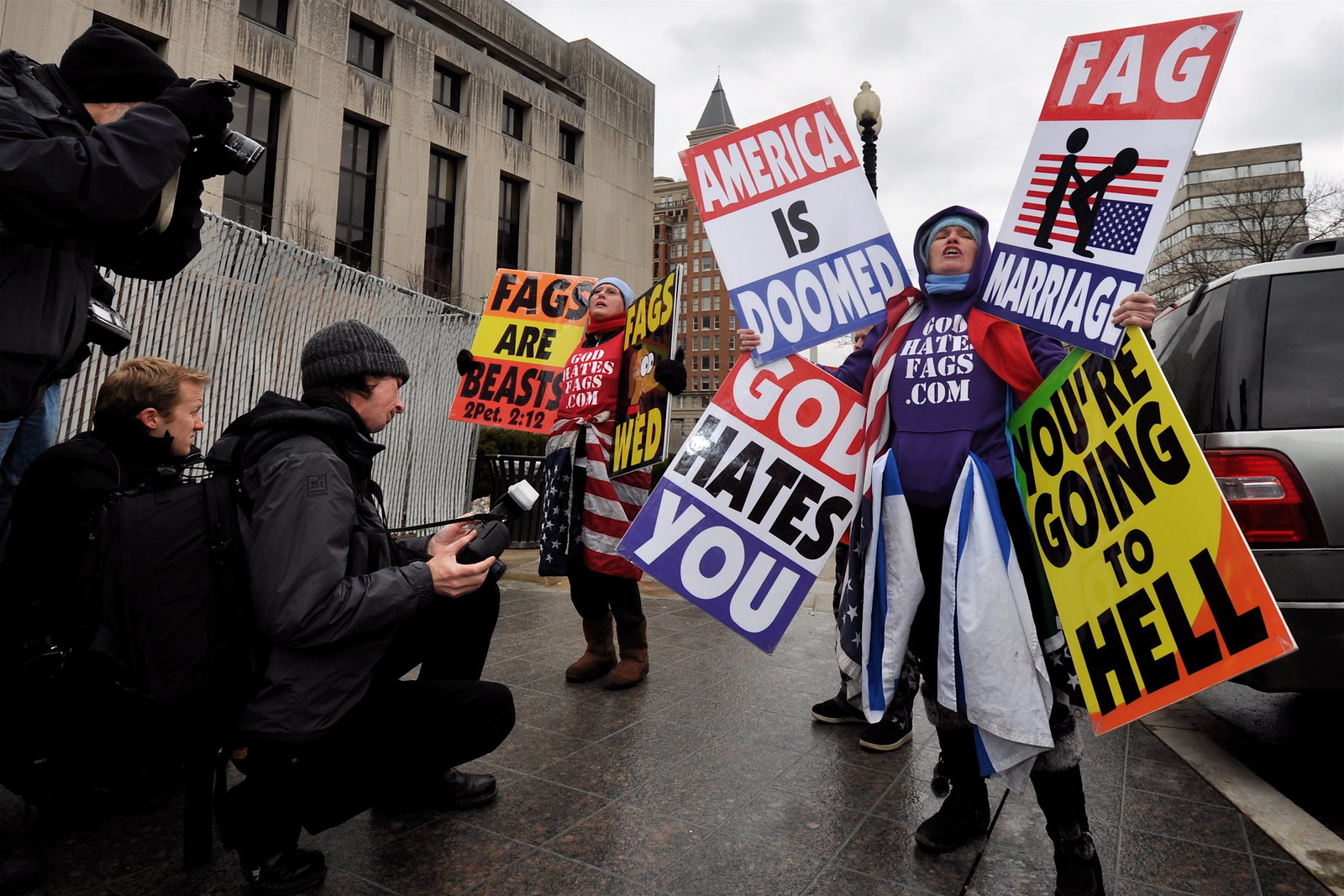In this photograph taken on a cloudy, overcast day, six individuals are depicted on a city street engaged in a protest. The primary focus is on two protesters positioned on the right side of the image, standing on a dark stone sidewalk near a car. The person in the front wears dark pants and a blue hooded sweatshirt with white text reading "godhatesfags.com" and an American flag draped around their neck. In their hands are four signs with messages including "America is doomed," "God hates you," and others with derogatory phrases. Behind this individual stands another protester dressed in dark pants and boots, a red hooded sweatshirt with the same controversial URL, and an American flag tied around their waist. This person also holds inflammatory signs reading "fags are beasts" and "fags wed."

On the left side of the image, a group of people, mostly dressed in black, are seen photographing the protesters. The backdrop features several multi-story buildings, a large stone building with tall windows, a fence, and a black lamppost. The sky is a mix of grey and white, adding to the gloomy atmosphere. A car is partially visible on the right edge of the photo, contributing to the urban setting.